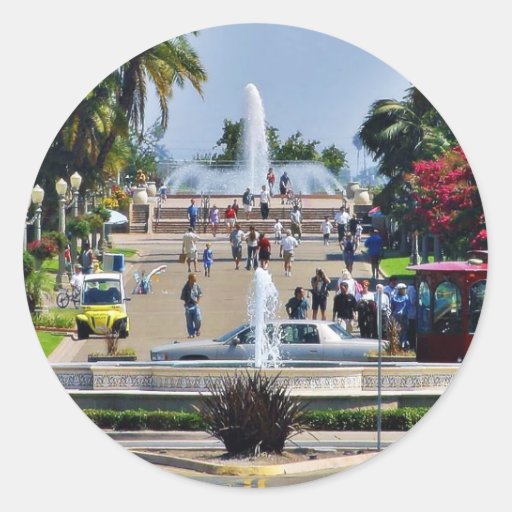This image, centrally framed within a white, eggshell background, captures a vibrant outdoor scene that appears to be a park or a popular public space, possibly in Southern California. The circular photo is filled with lively details: two water fountains grab attention, with the nearer one shooting white sprays of water and a larger one further back. The park is bustling with people, all dressed in shorts, suggesting it's a sunny, pleasant time of year.

Numerous palm trees and a striking tree with bright pink flowers create a tropical, colorful atmosphere. Among the crowd, various vehicles are spotted, including a silver sedan, a yellow golf cart, and part of a red trolley behind the car. A cyclist also navigates the clean, well-maintained sidewalk lined with lampposts. The scene brims with vibrant hues – grays, blues, greens, browns, whites, reds, yellows, purples, and pinks – making it visually rich and indicative of a potential vacation destination.